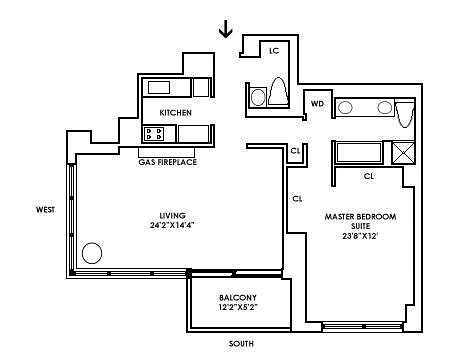This digital mock-up showcases a detailed blueprint of a small house or apartment, rendered in black lines on a white background. The outer structure is demarcated with double lines, while single black lines outline the internal rooms.

On the leftmost side, the living room spans 24' 2" by 14' 4", featuring a gas fireplace in the upper section and an intriguing unlabeled round circle in the lower left corner. Adjacent to the living room, down and to the right, lies a balcony measuring 12' 2" by 5' 2". Further right, the master bedroom suite extends 23' 8" by 12". Positioned above the master bedroom is a room that appears to be a bathroom, though it lacks explicit labeling. At the very top, the kitchen is situated next to an area marked "LC," which is possibly another bathroom.

The main entrance is centrally located at the top of the blueprint, indicated by a black arrow pointing inward. The exterior boundaries to the left and bottom of the house are labeled as West and South, respectively. While the drawing is monochromatic and basic in its representation of amenities like the fireplace and kitchen stove top, it offers a precise and functional layout of the home's living spaces.